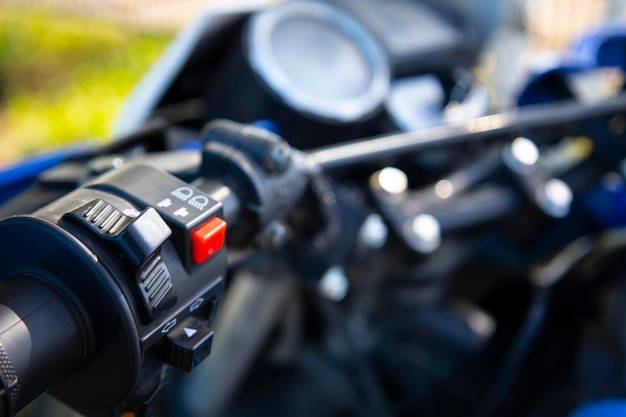This is a detailed close-up photograph of the left handlebar of a motorcycle, focusing specifically on the headlight control area. The image highlights a black handlebar, with a prominent red button that serves to operate the headlights. Above this red button are two symbols resembling jellyfish, indicating the low and high beam settings. Adjacent to the red button on the left is a black switch, though its function isn't clear. Below the red button sits another black button, which features a white arrow and two additional white arrows above it, pointing left and right, likely for controlling the turn signals. The rest of the motorcycle is blurred and obscured, but a circular speedometer, several bolts, and a wire running from the handle are faintly visible. The motorbike's body appears to be black and blue in color.